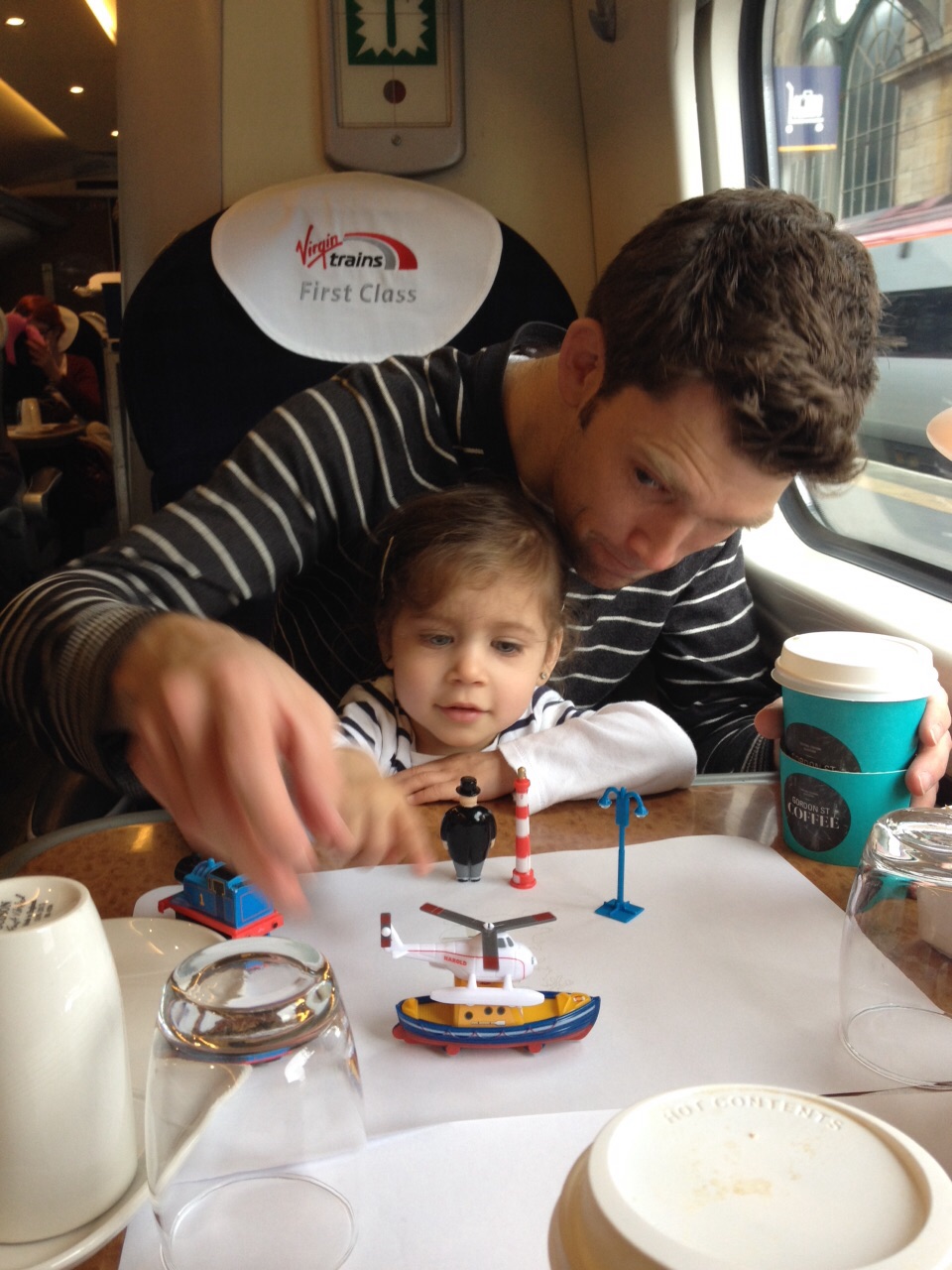A detailed image of a father and his young daughter, approximately two to three years old, sitting in a Virgin Trains First Class compartment. Both of them have brown hair and are dressed in matching black-and-white striped t-shirts. The father, who has brown hair, is holding a coffee cup in his left hand while engaging with toys on the table in front of them, using his right hand. The toys include a helicopter, a small figure with a lantern, and possibly some Lego pieces featuring a lighthouse. The table is cluttered with various items including two glasses, a coffee cup with green packaging, another upside-down coffee mug, and some additional containers. Through the window to their right, there is a blurred view of another train and a stone train station building in the background. The overall color palette of the scene includes shades of black, white, blue, and brown. The father and daughter are focused intently on the toy, creating an intimate and playful moment amidst the comfortable setting of the train.